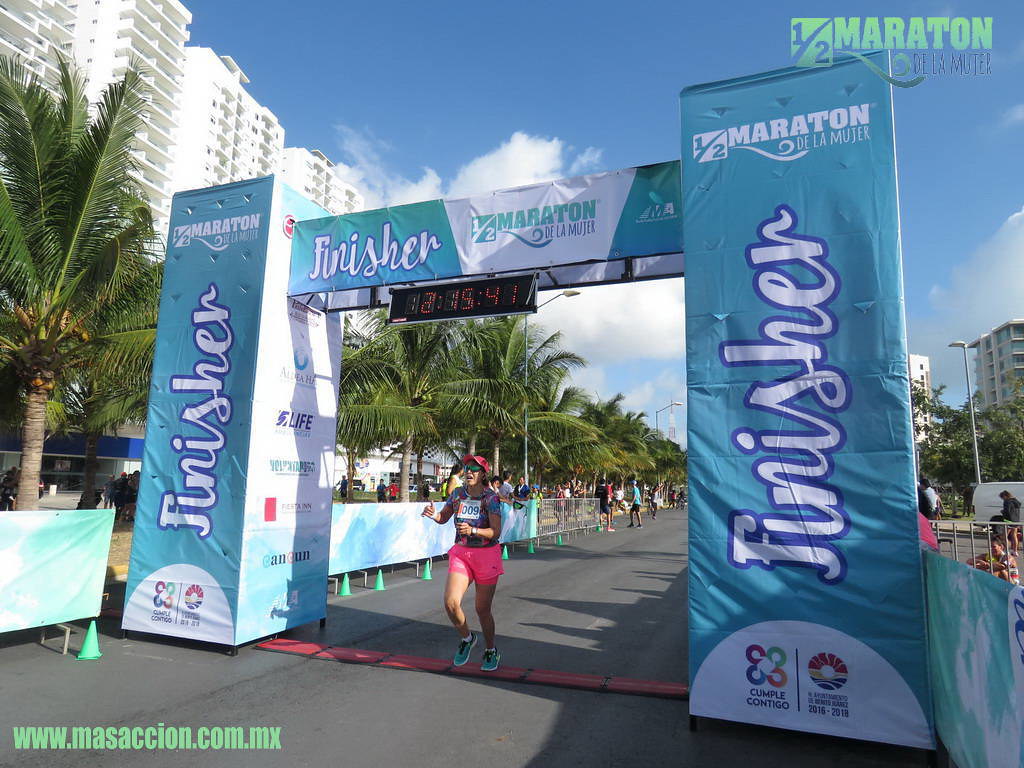This vibrant outdoor photograph captures the triumphant moment of a marathon runner crossing the finish line under a clear blue sky. The scene is set at the Half Marathon de la Muerte, as indicated by a green watermark in the upper right corner. In the lower left, the website www.massaccion.com.mx is visible. The timed clock above the runner shows her impressive finish of 2 hours, 15 minutes, 41 seconds.

The runner, a woman clad in pink shorts, a T-shirt, and a race bib, completes her journey under a prominent banner that reads "Furnisher," the event’s sponsor. She is also sporting a hat and sunglasses. Palm trees line the race course, adding a touch of tropical ambiance, and there is a sparse but supportive group of onlookers on the roadside cheering her on. Behind her, other runners make their way towards the finish under the blue-and-white banners. Tall white and blue buildings, probably hotels, rise on the left side, framing this moment of achievement in an idyllic setting.